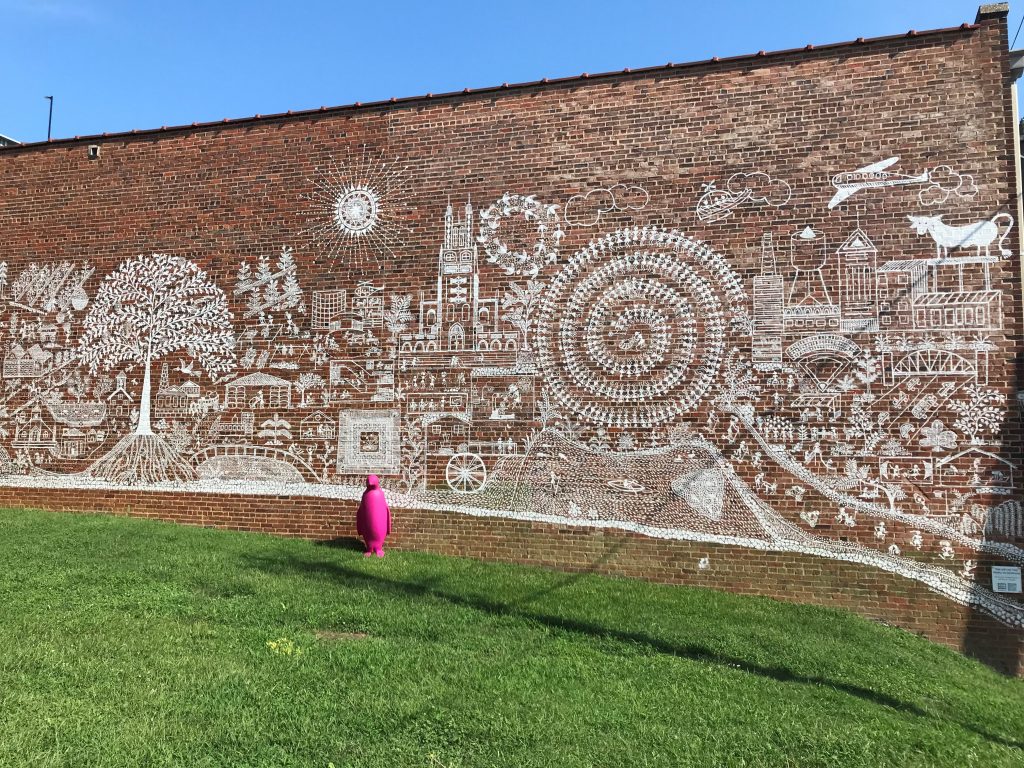This image depicts a sunny outdoor scene dominated by a red brick wall adorned with an intricate white mural. The mural features a variety of detailed drawings, primarily showcasing a townscape with buildings, trees, and their roots. Prominent elements include a large spiral pattern surrounded by floral designs, as well as whimsical touches like a cow standing atop a building in the upper right-hand corner, an airplane flying above, and little clouds near what appears to be the sun in the sky above. The mural also includes wheels at the bottom and a house. The sky above the wall is clear and blue, with more expanses of sky visible on the left side of the image. In front of the wall, standing on the green grass, is a tall plastic penguin colored entirely in pink, adding a quirky touch to the mural scene.